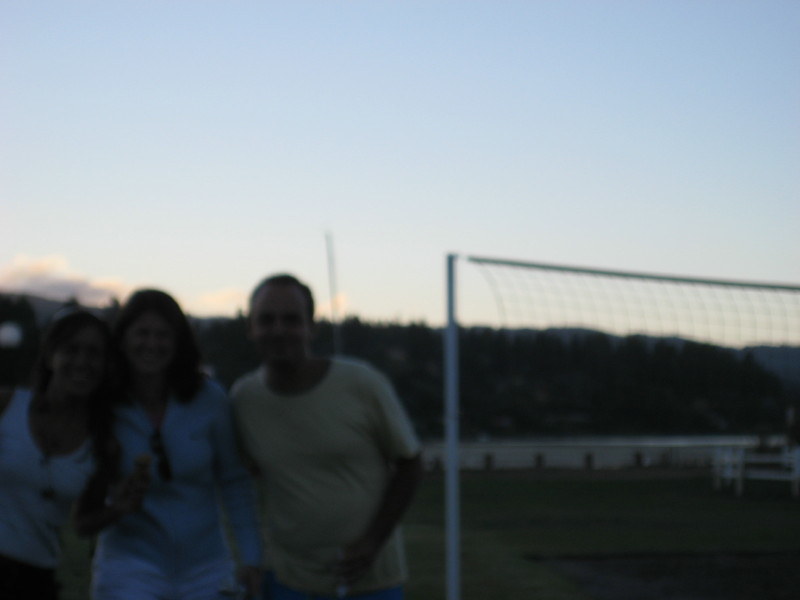An old, slightly blurry photograph captures a moment outdoors in what appears to be a field. In the background, just a few feet away, stands a large sports net, possibly for tennis or volleyball, accompanied by a light pole and a small dog bench, hinting at a recreational setting. 

In the foreground, three people stand together: a young brunette woman wearing a blue shirt and matching blue shorts, and two older individuals who bear a striking resemblance to her. The older woman, who looks to be in her early 40s, has dark hair and is dressed in a white tank top. On the other side of the young woman stands an older man, also seemingly in his early 40s, with a receding hairline and a light yellow shirt. Although it is not certain, the trio's strong family resemblance suggests that the older couple might be the young woman's parents.